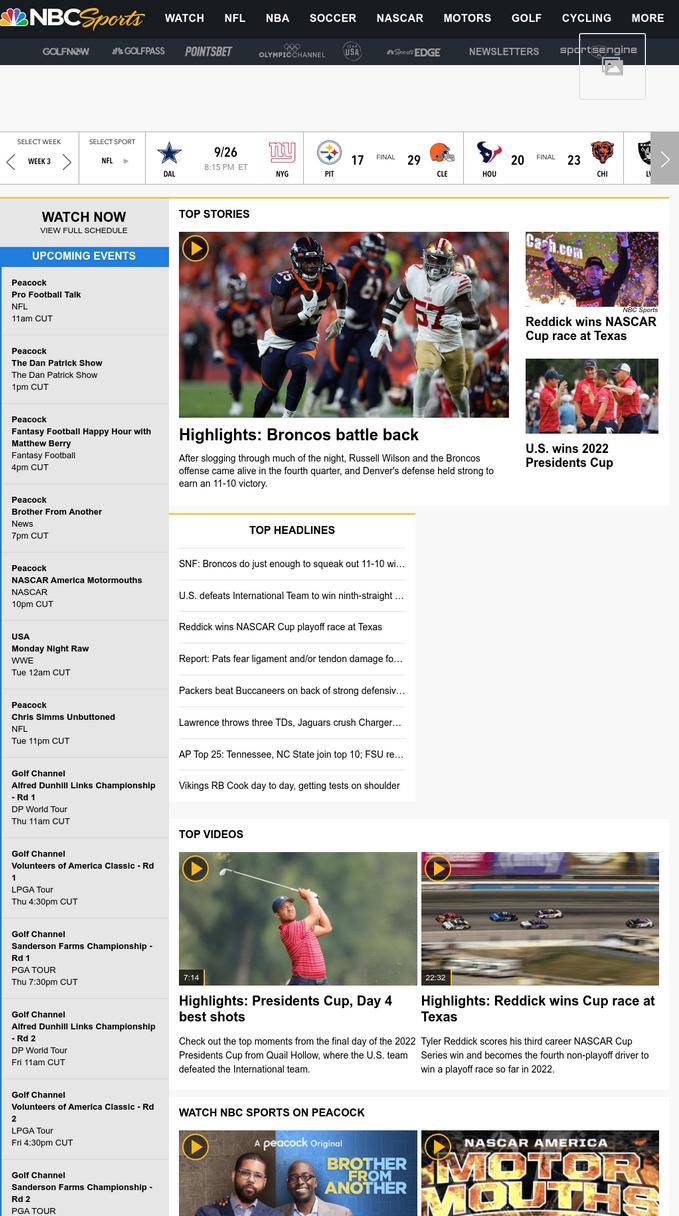This image captures a screenshot of the NBC Sports website. Dominating the top portion is the iconic NBC rainbow peacock logo, followed by the words "NBC Sports" in a striking white and yellow font. Below the header, the top menu bar prominently displays quick links to various sports categories such as NFL, NBA, Soccer, NASCAR, Motors, Golf, and Cycling.

Beneath this primary menu, there is a secondary menu that features smaller logos, which seemingly represent specific channels or related services. These include Golf Pass, Points Bet, Newsletters, and Sports Engine, among others, though some are too small to easily identify.

Mid-screen, there are scores of recent games highlighted, detailing match-ups such as Dallas versus New York as an upcoming event and the results for Pittsburgh versus Cleveland. Adjacent to this is an "Upcoming Events" section that appears to list specific upcoming programs or games rather than a generic menu.

Further down, the "Top Stories" section showcases various highlighted news articles. One of the headlines visible reads "Broncos Battle Back," displayed alongside other notable stories and highlights. The overall design is clean with a light gray background, black text, and blue and yellow accent colors, presenting information in a visually engaging yet detailed manner.